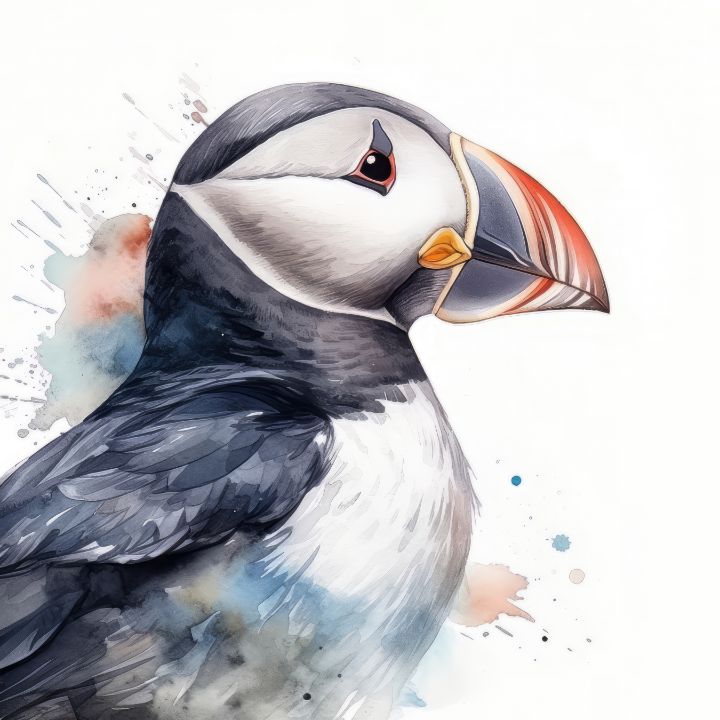The detailed piece of art depicts a relatively large bird that resembles a penguin but also has features hinting at a toucan. Executed in a watercolor-like technique, the bird has a distinctively large, multicolored beak adorned with stripes, featuring orange, grey, blue, red, and white. The beak's nostril is tinged with orange. The bird's eye is primarily black, adorned with grey and orange details, and a small white spot that adds depth and emotion, suggesting a somewhat sad expression. The plumage is richly textured: the head is predominantly black on top with white on the cheeks, transitioning into black over the back and under the neck. The chest feathers are predominantly white, blending into blue and grey further down the body. In the background, vibrant splashes of pink, red, blue, light blue, green, and orange create an abstract, dynamic texture, adding depth and a sense of spontaneity to the artwork. The overall effect combines meticulous detailing of the bird with an expressive and colorful background, enhancing the visual interest and emotional tone of the piece.